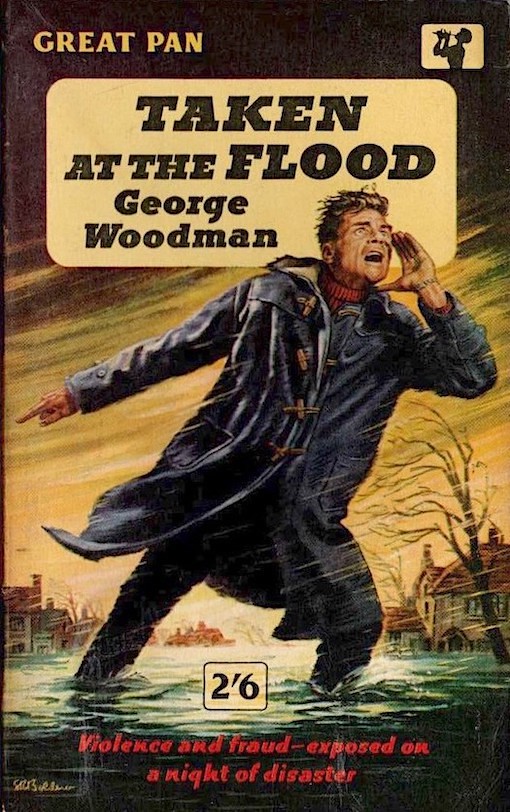This image appears to be the cover of a book titled "Taken at the Flood" by George Woodman, published by Great Pan. The cover features a dramatic drawing rather than a photograph. In the top left corner, the publisher's name, "Great Pan," is prominently displayed. There is a logo in the top right corner, depicting a woman playing a trumpet or similar instrument. The title "Taken at the Flood" is set in black text against a yellow background, with the author's name, George Woodman, following beneath it. Below this, in red text, it declares, "Violence and Fraud Exposed on a Night of Disaster."

The scene illustrated shows a flooded environment with water rising to about ankle height. In the foreground, a man, who appears to be a white male with short dark brown hair, stands in the rising water. He is wearing a blue rain jacket over a red sweater, paired with black pants. The man is leaning into the wind and pointing while calling out, his hand cupped around his mouth. The background is chaotic, with trees and several houses barely above the water line, emphasizing the severity of the flood and the storm.